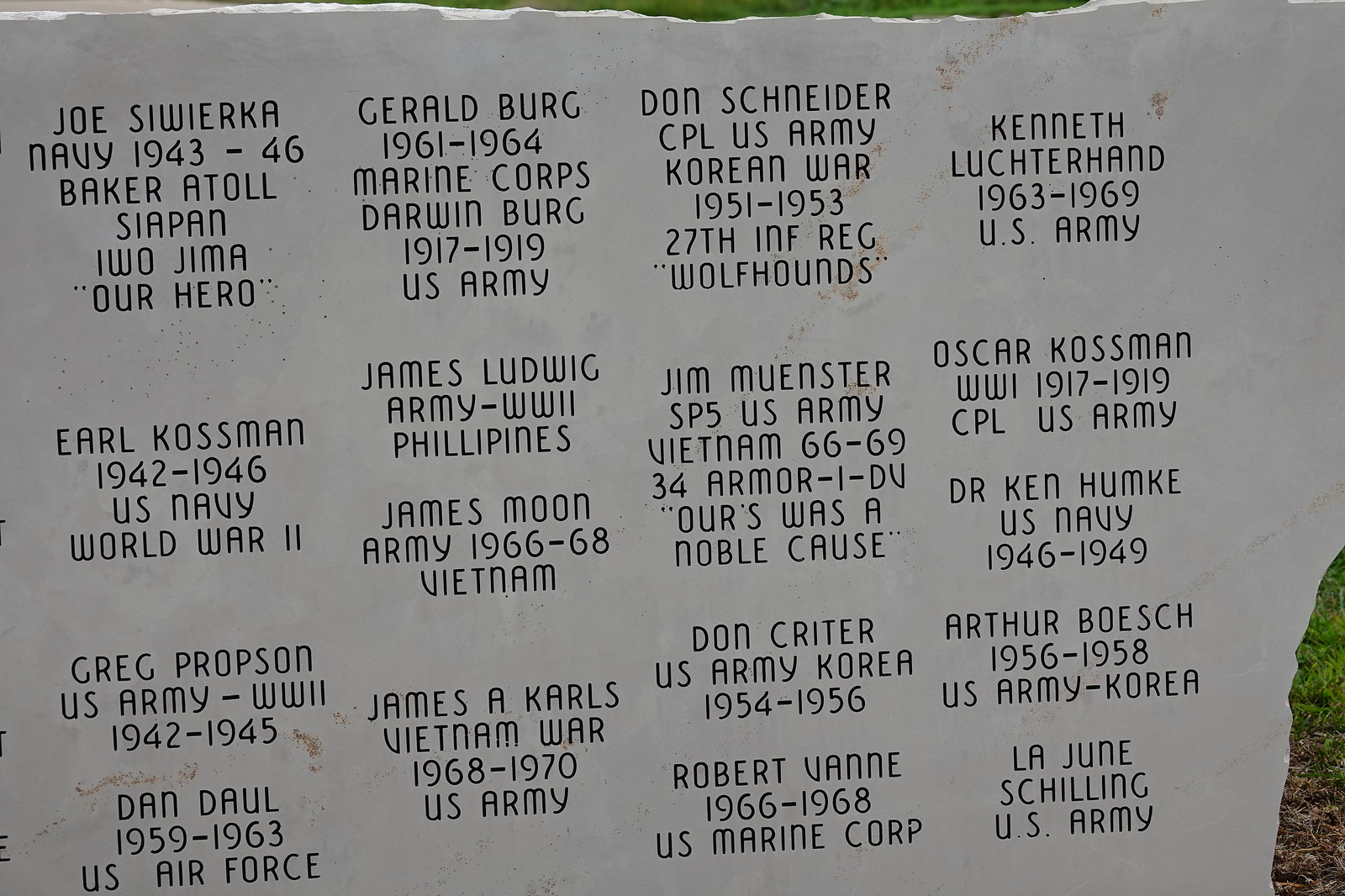In this horizontally aligned rectangular image, an outdoor setting is depicted, marked by visible grass patches in the lower right-hand corner and along the top center. Dominating the scene is a gray, potentially breakable, rock or cardboard-like material, seeming uneven at the top with a broken piece at the bottom right. This central object features meticulously printed or carved black-lettered names of military personnel, each accompanied by their service branch, service years, locations served, and occasionally a personal quote or designation. For instance, the top row includes names like "Joe Swierka, Navy, 1943-1946, Baker Atoll, Saipan, Iwo Jima, 'Our Hero'" spanning five lines. Similarly, "Gerald Berg, 1961-1964, Marine Corps" accompanies other names in the first row, and the pattern continues across three rows totaling approximately twelve names. The structure and details suggest this could be a commemorative war monument, present in a serene grassy field under daylight, honoring the service and sacrifices of these military members. The overall colors are predominantly gray, black, green, and brown. The image accentuates the detailed inscriptions and the solemnity of the memorial.